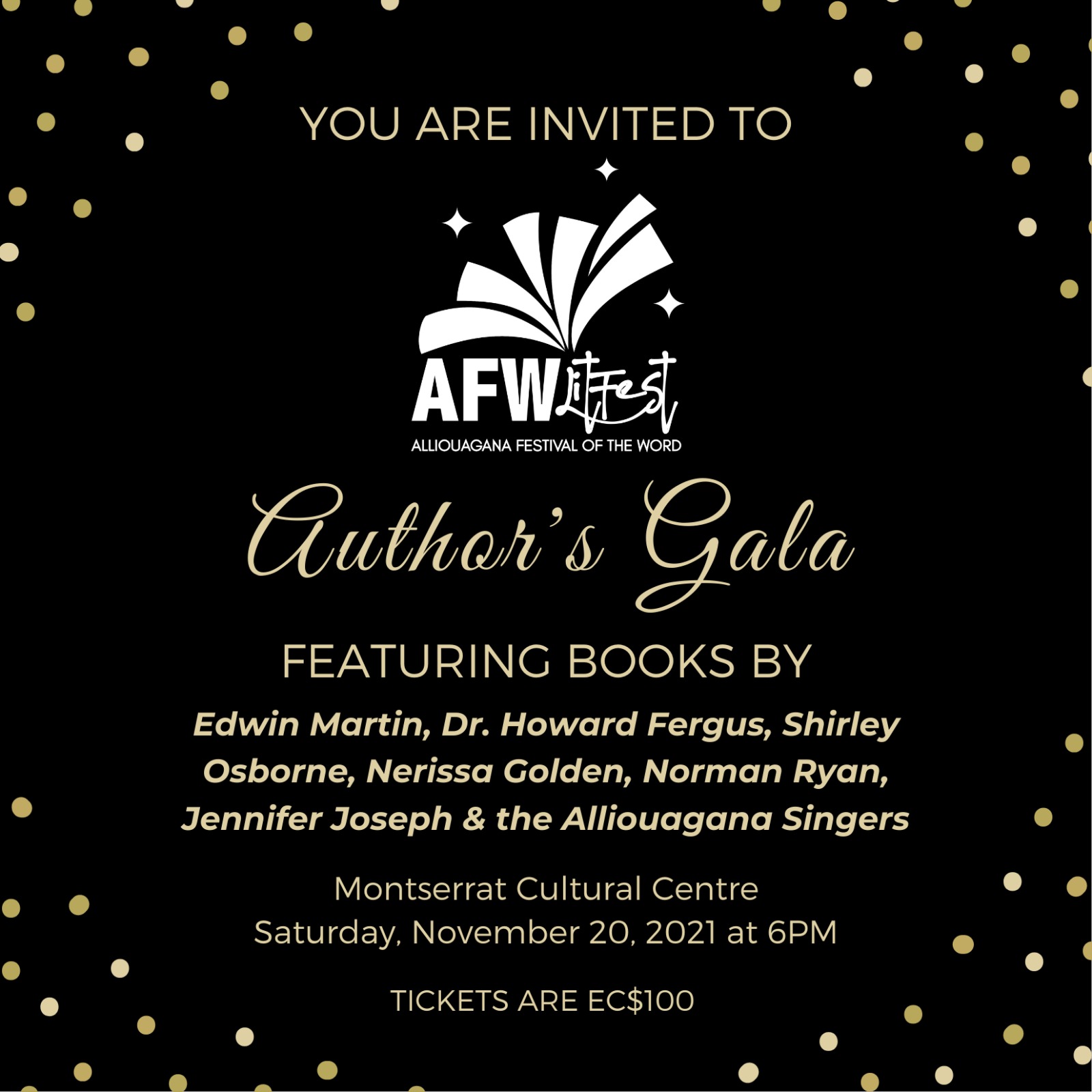This elegant invitation flyer features a sleek black background adorned with shimmering gold confetti in all four corners. At the top, bold white text announces, "You are invited to AFW LifeFest," followed by "Ali Oaga Ghana Festival of the World" in a smaller font. Below, the invitation highlights the "Authors Gala," showcasing books by Edwin Martin, Dr. Howard Fergus, Shirley Osborne, Nerissa Golden, Norman Ryan, and Jennifer Josen, accompanied by a performance from the Ali Oaga Ghana Singers. The event details are meticulously listed at the bottom: "Montserrat Cultural Center, Saturday, November 20th, 2021 at 6pm," with tickets priced at $100.